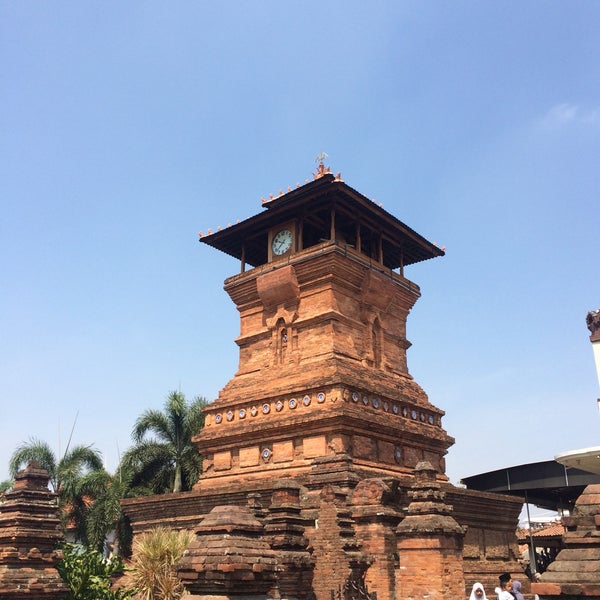The image captures a tall, clay-colored structure with a blend of historical and architectural significance, possibly located in Asia. The building, made of stone or brick, features a golden-brown hue. It has a distinct flared roof supported by a dozen pillars and topped with several gold emblems. A prominent clock with black hands is situated just beneath the roof, displaying a time close to either 10 till 8 or 10:40. Ornamental circular designs adorn its midsection, while its overall boxy, ancient appearance suggests significant historical craftsmanship. In the background, the sky is mostly clear with blue and white colors, complemented by wispy clouds. Tall trees with palm-like leaves are visible to the left. Additional buildings with gray coverings are seen to the right, and there are three figures in the lower right corner, likely artists capturing the scene.